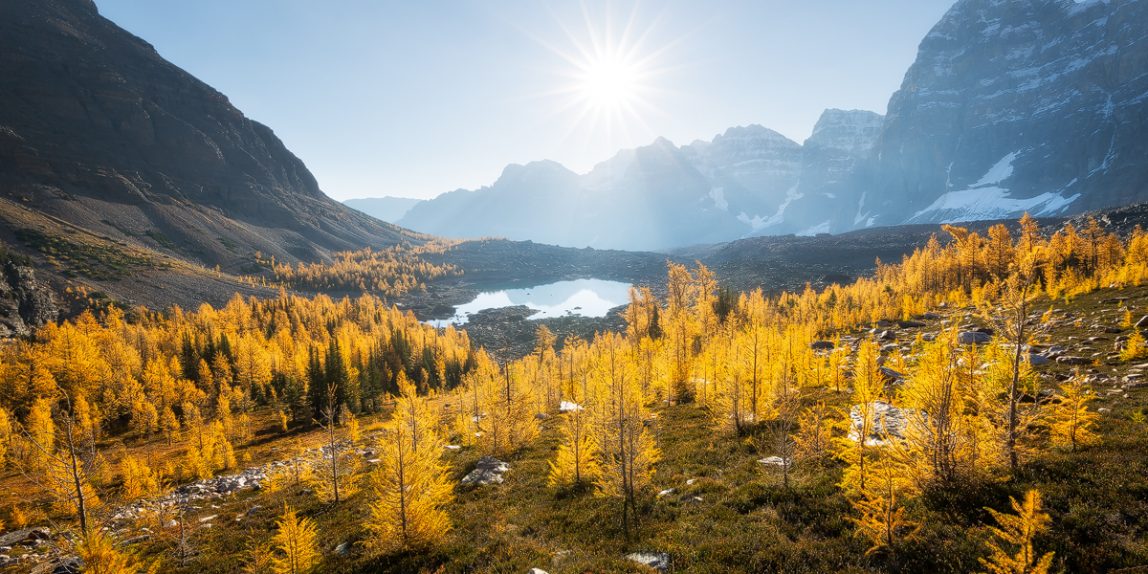This breathtaking image captures a scenic mountain panorama, showcasing a striking blend of autumnal and wintry elements. In the foreground, a hillside adorned with green growth and uniformly yellow, conifer-like trees stretches out, their vibrant leaves extending all the way to the ground. At the heart of the scene lies a serene mountain lake, its surface mirroring the rugged terrain and brilliant sunshine above. Framed by imposing mountains on both sides, the lake is cradled in a valley that offers a lush contrast against the surrounding rocky slopes. The mountains to the left are barren, while those on the right display patches of enduring snow. Beyond these, distant snow-capped peaks rise, completing the majestic backdrop. Dominating the sky, a radiant sun emits sharp, triangular rays, illuminating the bluish-gray expanse above. This harmonious composition of golden autumn foliage, reflective waters, and towering snow-dusted mountains is a testament to nature's mesmerizing beauty.